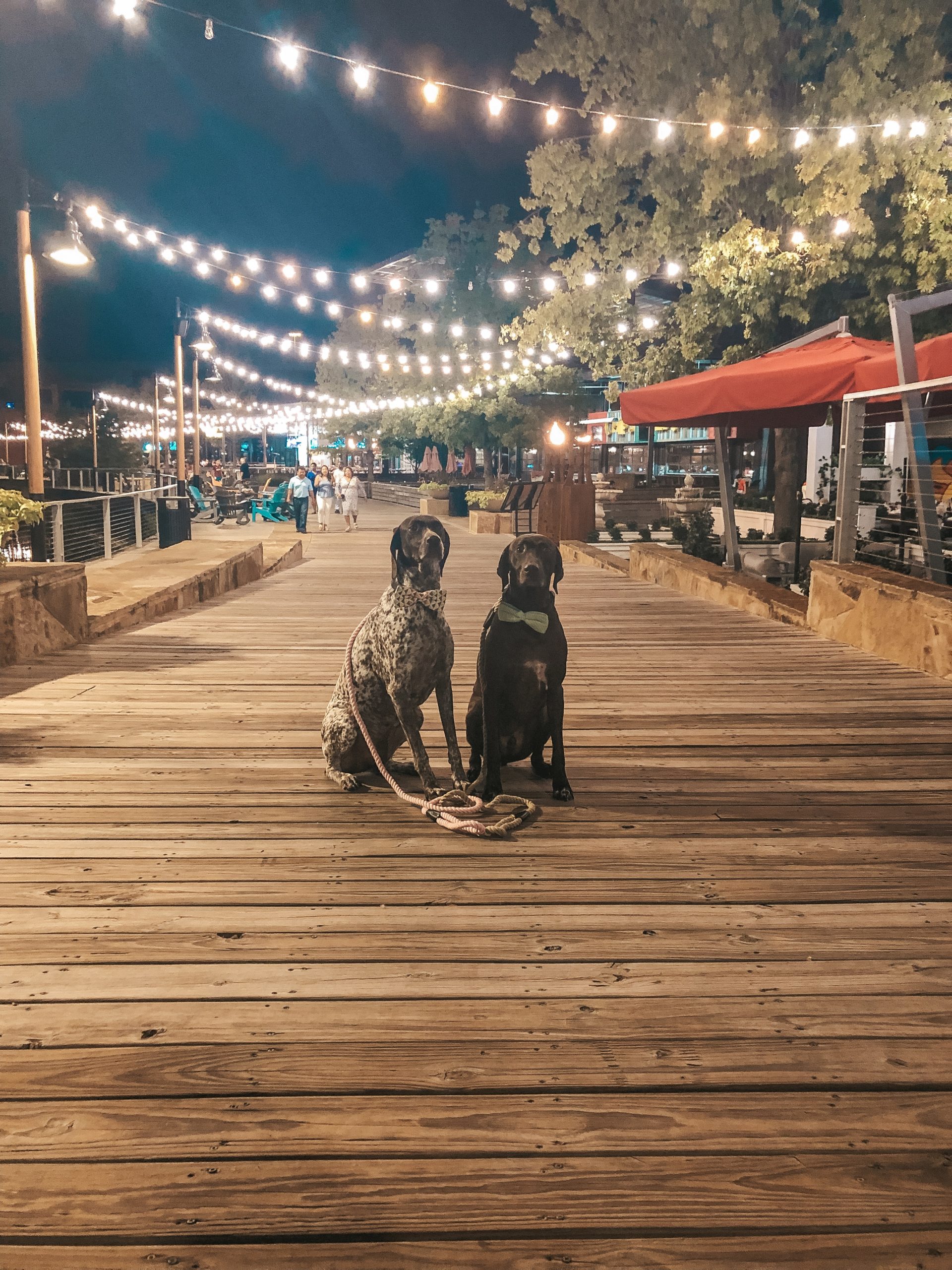In this enchanting evening outdoor scene, the sky transitions from a deep dark blue at the edges to a medium midnight blue towards the center. The serene atmosphere is illuminated by light fixtures mounted on poles that line the left side of the boardwalk-style walkway. The path itself, constructed of light wooden planks, is bordered by a railing on the left, where it seems to overlook a body of water below.

On the right side, there's a lush row of trees, and various eateries offering cozy seating areas for visitors. The entire walkway is festively adorned with string lights, casting a warm, inviting glow over the scene. People stroll leisurely in both directions, adding to the bustling yet calm ambiance. 

Amidst the crowd, two large dogs catch the eye: a German Pointer wearing a charming white bow tie with red polka dots and a long pink leash, and a Labrador with a light green bow tie and a black lead rope. The dogs, with their elegant bow ties and poised manners, become the delightful focal point of this lively, picturesque evening setting.